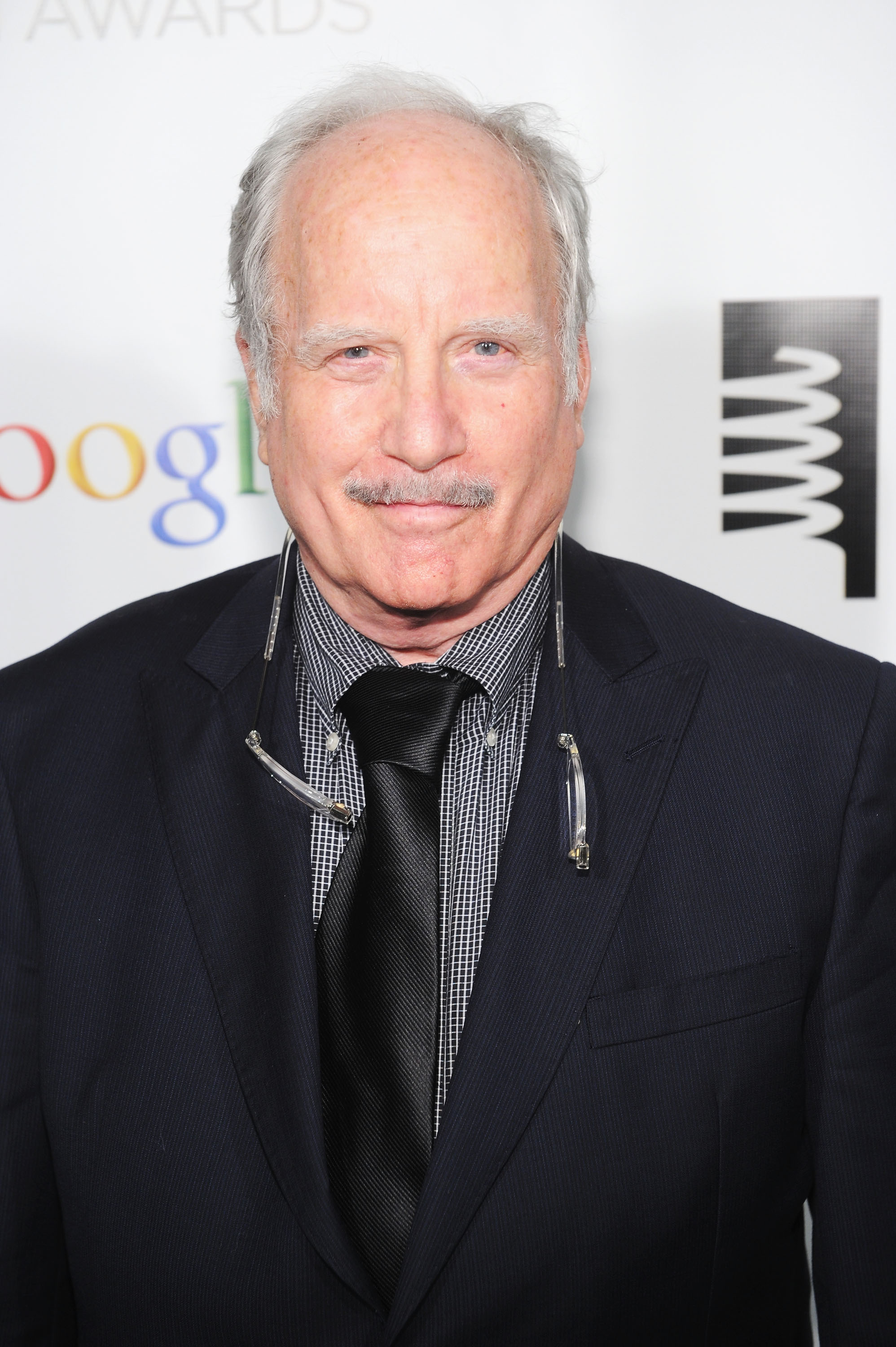The image is a detailed close-up photograph of Richard Dreyfuss. Centered in the photo, he looks directly forward with a slight smile, revealing a square chin. Dreyfuss sports short, silver hair that's thin on top and thicker on the sides, along with matching gray eyebrows and a thin gray mustache. He is dressed in a dark blue sports jacket paired with a black tie, which is not tied neatly. His shirt underneath features a pattern of black and white specks. Around his neck hangs a pair of reading glasses that clasp together when worn. The photograph cuts off around his stomach level and his arms are mostly down by his sides, with the left arm partially visible off the bottom and right side of the picture. He is standing in front of a white wall displaying the Google logo to the left of his head and another black and white symbol to the right.